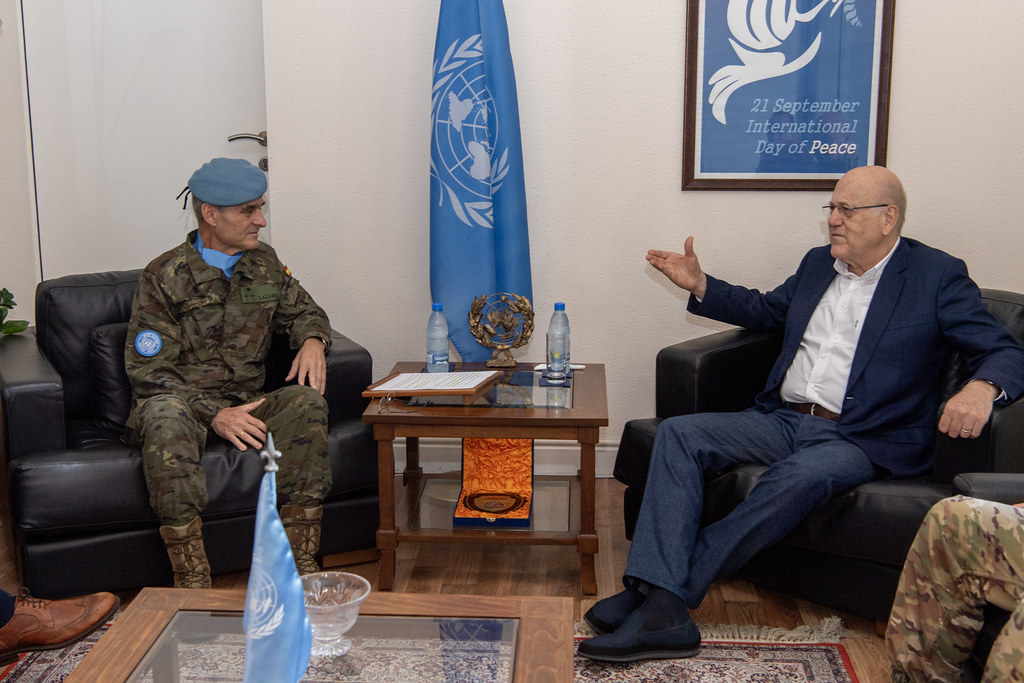In the photograph, two men are seated on black chairs, positioned centrally, engaged in a conversation. The man on the left is wearing a military uniform with camouflage green and brown colors, a blue t-shirt, and a blue beret adorned with the UN symbol on his sleeve. The individual on the right, appearing to be in his 60s, is dressed in a blue suit jacket, white shirt, blue jeans, and blue shoes. A coffee table, wooden-framed with a glass top, stands between them. This table holds two water bottles, a glass vase, papers, and a UN gold trophy featuring the iconic map and laurel wreath. Additionally, a side table nearby also bears two water bottles. Behind them, a large blue and white poster reads "21 September International Day of Peace," with 'Peace' highlighted in white against a darker blue background. Two flags, resembling NATO or the UN, are prominently displayed: one positioned between the two men and another placed on the coffee table. The scene exudes a formal atmosphere, likely related to the International Day of Peace as indicated by the poster text.